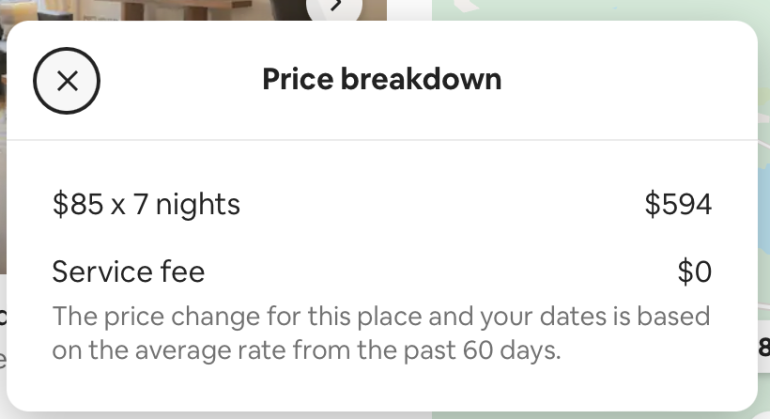In the image, there is a prominent white box overlaying a colorful background. The background, partially obscured, appears to show elements characteristic of a hotel room, such as a door and curtains on the top left. Within the white box, there is an X inside a circle located in the top-left corner.

Next to this symbol, black text reads "Price Breakdown." Beneath this, the pricing details are outlined: the cost is $85 per night for 7 nights, culminating in a total of $594, which is listed on the far right. A service fee section is included below, indicating a charge of $0.

At the bottom left, additional text explains that the price change is based on the average rate over the past 60 days, suggesting that the rates are variable. The overall design is clean, with black text on a white background, providing clear and organized pricing information, likely for a hotel or similar lodging service. To the right of the covered area, part of what seems to be a map is visible, possibly offering directions to the establishment.

In summary, the white box provides a detailed breakdown of accommodation costs, set against a partially visible background potentially depicting a hotel room setup.